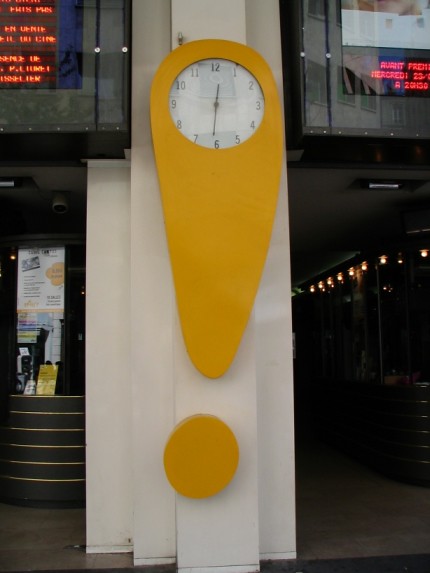This outdoor photograph captures a unique and abstract city street scene dominated by a distinctive clock designed in the shape of a large yellow exclamation point. The clock face, displaying the time around 12:30, is located at the top portion of the exclamation point, complete with black hands and numbers. The bottom of the exclamation point is a yellow dot. The clock is mounted on a protruding white post of a building, which consists of three layered sections. On the left side of the image, there's a window with some papers, and above the space is a digital display with wording in French. To the right, a dark hallway is illuminated by a series of lights along the top, disappearing into the distance. Red ticker signs flank each side of the scene, adding to the urban ambiance.